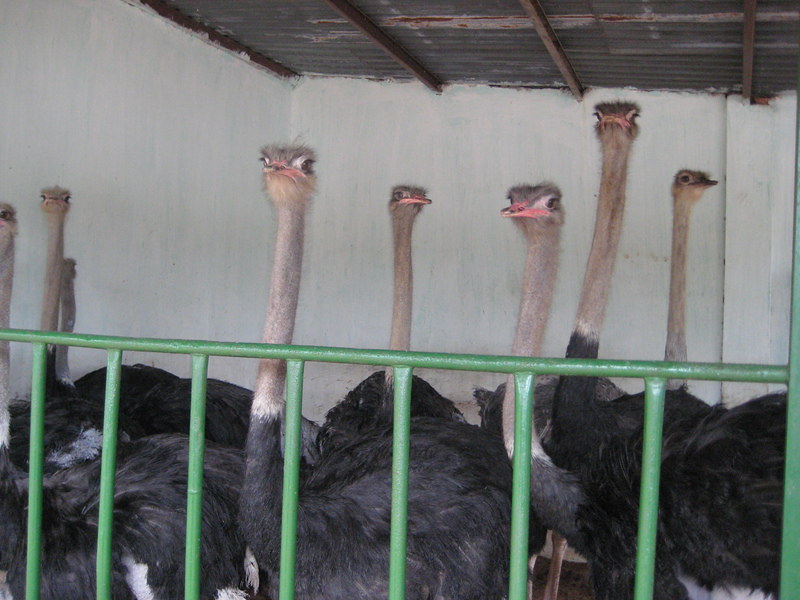This is a detailed photograph capturing numerous ostriches congregated in a confined pen, all appearing to look directly at the camera. The setting includes a contrasting dark wooden ceiling and a white wall, making the green metal fence in front of the birds quite prominent. The image showcases the ostriches' imposing stature, emphasizing their lengthy two-toned necks that are predominantly brown or gray, transitioning into light brown, with a distinctive thin white stripe below the neck which then meets their large black bodies dotted with sparse white feathers. Notably, their huge eyes exhibit a rather striking wide-eyed gaze complemented by large pink beaks. The space, which seems rather limited for these sizable creatures, accentuates their impressive height and collective curiosity as they stretch their necks, with one in the back particularly reaching its full length, creating a sense of unified observation.